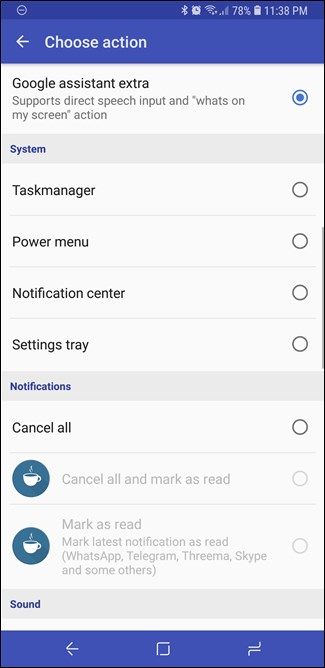A detailed caption for the described screenshot:

---

The screenshot captures a smartphone screen with a medium blue top border. On the right side of this border, in white font, the time is displayed as 11:38 PM, alongside icons for battery life (78% charged), wireless connection, Wi-Fi, an activated alarm clock, and Bluetooth.

Below this, the top border transitions into a slightly lighter royal blue. At the center, in white font, is the headline “Choose Action,” with a white left-pointing arrow on the left.

The main background of the screen is white, with very dark gray text, almost black. In the top left corner, it reads “Google Assistant Extra,” followed by a subtitle in lighter gray font: “Support Direct Speech Input and What’s on My Screen Action.” To the right of this text, there is a white circle with a blue dot inside, indicating an option has been selected.

A light gray line separates the next section labeled “System,” which spans the width of the screen. Under this section, listed items include “Task Manager” (written as one word), “Power Menu,” “Notification Center,” and “Settings Tray.”

Further down, another light gray line introduces the “Notifications” section. Beneath this, on the white background, is the text “Cancel All” written in light gray font. To the right is an oval-shaped, bluish-gray icon featuring a white coffee cup image. Below this, it reads “Mark as Read” (also in light gray font), followed by the description in parentheses: “Mark Latest Notifications as Read (WhatsApp, Telegram, Threema, Skype, and some others).”

The next section titled “Sound” is partially visible, indicating that scrolling is necessary to view its contents. 

Finally, the bottom border of the phone returns to the appealing shade of royal blue seen at the top.

---

This descriptive caption provides a comprehensive overview of the elements and layout of the smartphone screenshot.